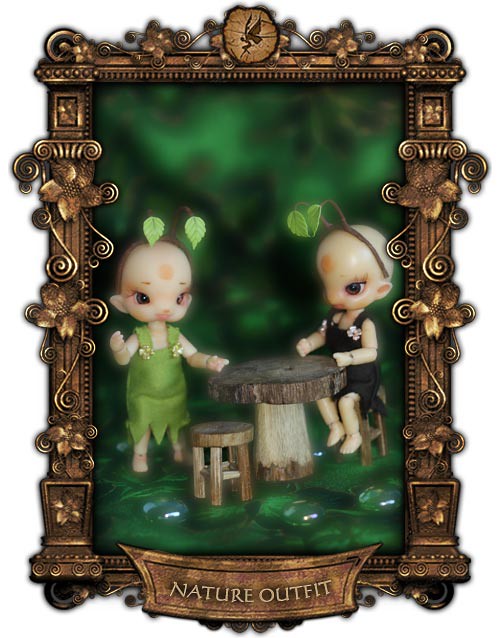The image is a detailed color photograph of a vintage collectible item, featuring an ornate brass-tone frame with a scroll effect and intricate, leaf-embellished designs reminiscent of fairy architecture and Greek pillars. At the top of the frame is an icon depicting a small winged fairy. The bottom of the frame houses a plaque with the phrase "Nature Outfit" inscribed on it. The image within the frame centers on two fairy-like dolls with humanoid features. These dolls have white plastic skin and small circles on their foreheads, resembling mystical markings. One doll is standing at a wooden table, crafted to look like a tree trunk, while the other is seated on a stool.

The standing doll is dressed in a dark green outfit adorned with a tiara made from twigs and leaves that resemble antennas. The seated doll wears a black dress and a black headband, with oversized eyes gazing downward. Both figures have a whimsical and ethereal appearance and are situated against an out-of-focus, forest-like background filled with green leaves and natural elements, enhancing the enchanting woodland theme.